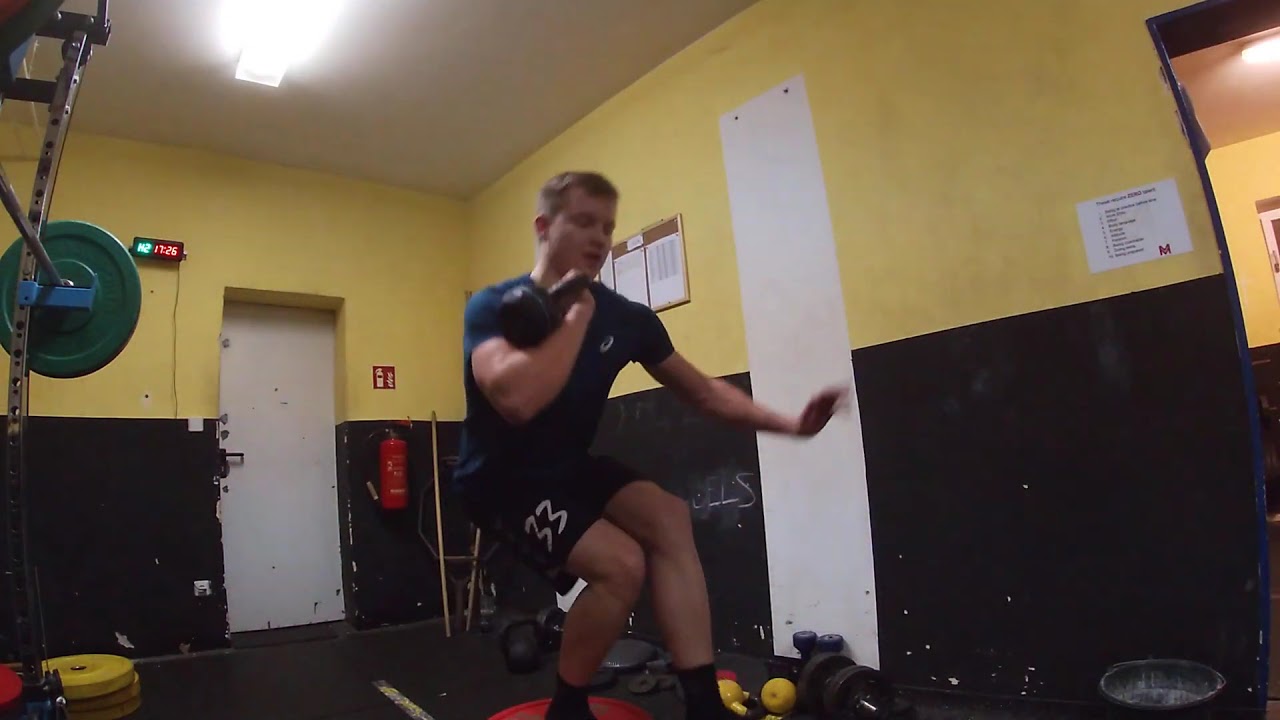The image captures a rundown, indoor gym, characterized by its black and yellow walls, with the paint visibly worn down. The horizontal, full-color photograph does not feature any border. In the background, a white door equipped with several locks stands centrally, flanked by a red fire extinguisher on one side and a digital clock displaying 17:26 on the other.

The focal point is a young Caucasian male with light brown hair, dressed in a blue short-sleeved t-shirt, blue shorts marked with the number 33, and dark socks. He appears to be mimicking a shot put stance, possibly practicing for a shot put competition. His left arm extends down at a 45-degree angle, while his right arm is bent with a kettlebell resting on his forearm near his chin. Surrounding him is standard gym equipment, including weights such as dumbbells and small free weights scattered on the floor. To his left, a barbell with green weights is mounted on the wall. The room features typical gym elements, contributing to the overall atmosphere of an old and used facility.